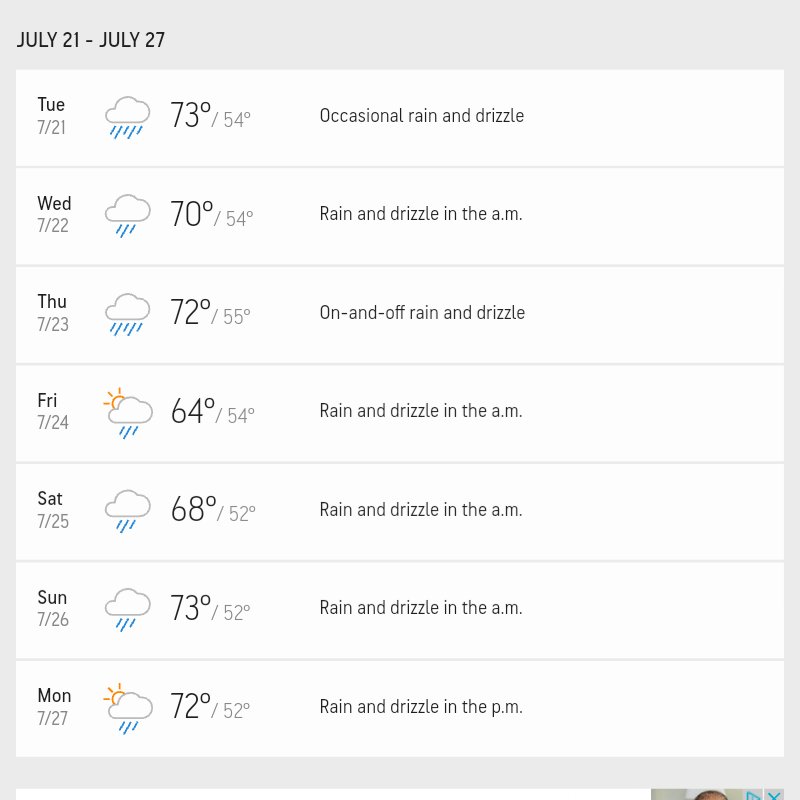The screenshot displays a section of a website with a light gray background. The layout features a thicker border at the top, thinner borders running down the left and right sides, and a border at the bottom that is slightly thicker than the sides but not as thick as the top.

At the top left of the screenshot, the text "JULY 21 TO JULY 27" is prominently displayed in capital letters. Below this heading are seven white rectangular panels arranged vertically. Each panel represents a day of the week with a weather forecast.

1. **Tuesday, July 21 (TUE 7-21)**:
   - Icon: Cloud with rain
   - Temperature: 73°F / 54°F
   - Description: Occasional rain and drizzle

2. **Wednesday, July 22 (WED 7-22)**:
   - Icon: Cloud with rain
   - Temperature: 70°F / 54°F
   - Description: Rain and drizzle in the a.m.

3. **Thursday, July 23 (THU 7-23)**:
   - Icon: Cloud with heavier rain
   - Temperature: 72°F / 55°F
   - Description: On and off rain and drizzle

4. **Friday, July 24 (FRI 7-24)**:
   - Icon: Partially sunny with a cloud and rain
   - Temperature: 64°F / 54°F
   - Description: Rain and drizzle in the a.m.

5. **Saturday, July 25 (SAT 7-25)**:
   - Icon: Cloud with rain
   - Temperature: 60°F / 52°F
   - Description: Rain and drizzle in the a.m.

6. **Sunday, July 26 (SUN 7-26)**:
   - Icon: Cloud with rain
   - Temperature: 73°F / 52°F
   - Description: Rain and drizzle in the a.m.

7. **Monday, July 27 (MON 7-27)**:
   - Icon: Sun partially covered by a cloud with rain
   - Temperature: 72°F / 52°F
   - Description: Rain and drizzle in the p.m.